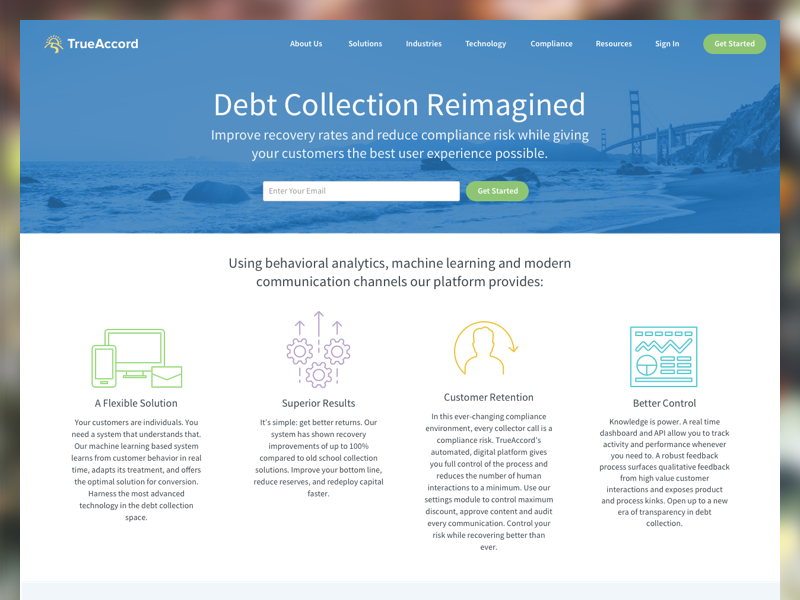**Website Overview: TrueAccord's Collection Reimagined**

The webpage features a background with a subtle blur effect, enhancing focus on the central content. The header area is dominated by a dark blue bezel, prominently displaying the company's logo: a stylized yellow sun with radiating lines above a flowing yellow stream. Adjacent to the logo, the company name "TrueAccord" is displayed in bold white text. To the right, several navigation tabs are visible in regular white text, including "About Us," "Solutions," "Industries," "Technology," "Compliance," "Resources," and "Sign In." At the far right, an oval-shaped lime-green button with white text encourages visitors to "Get Started."

**Main Content Area and Call-to-Action:**

Centered in the page, bold white text reads, "Collection Reimagined," followed by a subheading in regular white text stating, "Improve recovery rates and reduce compliance risk while giving your customers the best user experience possible." Beneath this is a rectangle with a white background and gray text, prompting users to "Enter your email." To the right is another lime-green oval button with white text declaring, "Get Started."

**Technological Advantages:**

Below the main call-to-action section, a large light gray area describes the platform's technological benefits in black text:

1. **Behavioral Analytics, Machine Learning, and Monitoring Communication Channels:** 
   - The left side features a computer, tablet, and envelope icon in lime green and black text promoting "A Flexible Solution." 
   - It details that the platform understands customers as individuals and adapts in real-time using machine learning for optimal conversion.

2. **Superior Results:** 
   - Illustrated with three interlocked purple gears and upward arrows, the headline "Superior Results" is in bold black. 
   - The text emphasizes the system's efficacy, stating recovery improvements by about 100% compared to traditional methods, aiming to enhance the bottom line, reduce reserves, and accelerate capital redeployment.

3. **Consumer Retention:** 
   - The right side includes an orange silhouette of a person with a curving arrow, highlighting "Consumer Retention" in bold black. 
   - It explains that TrueAccord's automated digital platform minimizes compliance risk by reducing human interaction and offers full control through a settings module for auditing and improving communication.

**Superior Control and Feedback:**

- The section concludes with a focus on control, illustrated with various graphs, including a line graph and a pie chart:
   - The bold black text "Better Control" is followed by "Knowledge is Power," explaining that the real-time dashboard and API provide continuous activity and performance tracking. 
   - The feedback process aims to surface valuable insights from customer interactions, driving transparency and improvements in debt collection.